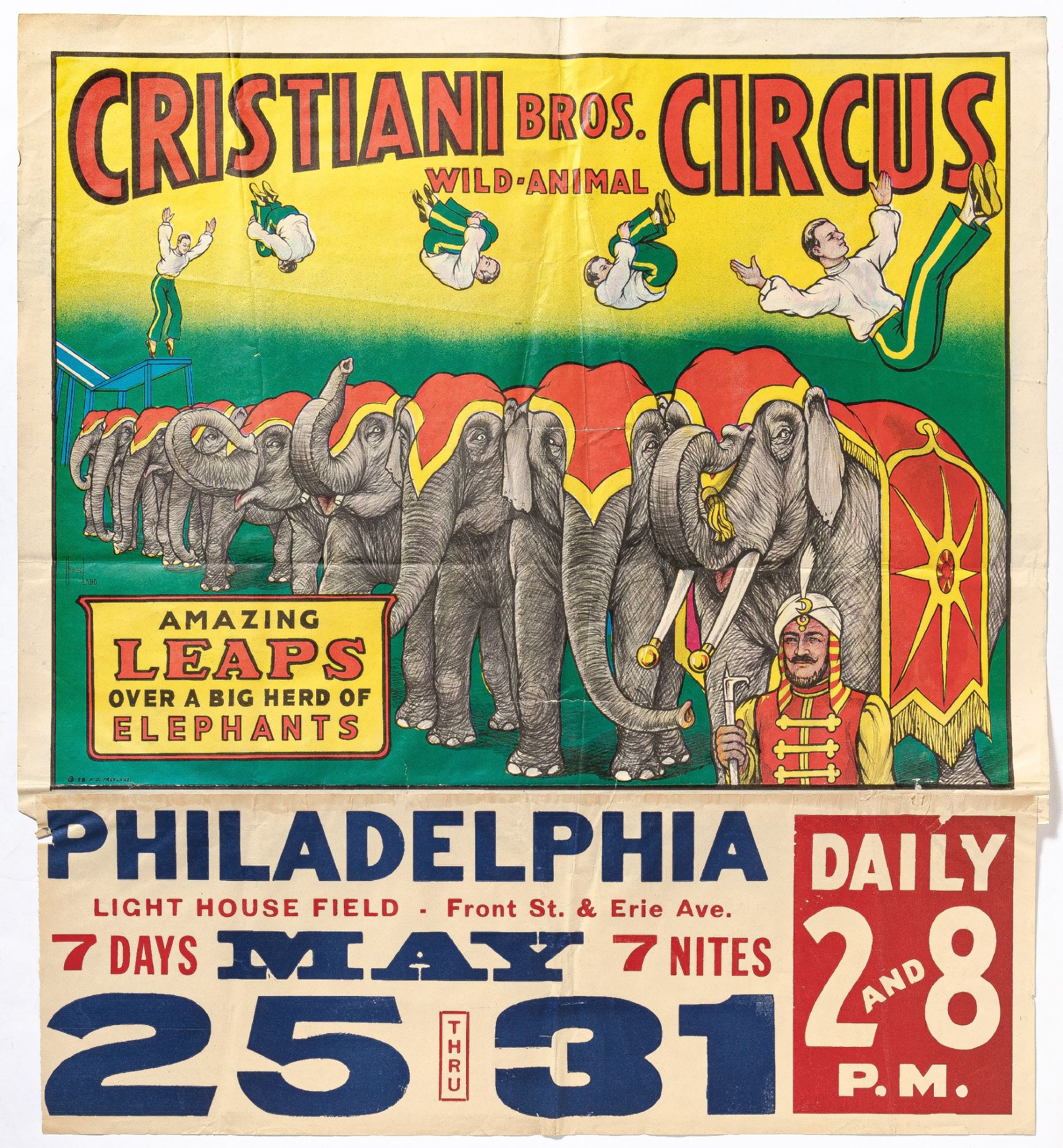This detailed, vintage poster advertises the Christiani Brothers Circus featuring wild animals. The poster is cream-colored and aged, with a distressed appearance. At the top, surrounded by a black border, the background transitions from yellow to green. Bold red letters announce "Christiani Brothers Circus Wild Animal." Below, there are five images showcasing an acrobat in mid-performance, dressed in a white shirt and green pants with a yellow stripe. He executes a series of somersaults, leaping off a blue board. Beneath this, the text proclaims "Amazing leaps over a big herd of elephants."

Centered on the poster, a line of elephants adorned in elaborate red and yellow costumes is featured, with decorative coverings draped over their sides and heads. At the head of the herd, a man with a white head covering, featuring a feather and a mustache, stands holding a guiding stick. He is dressed in an outfit matching the elephants' attire.

The event details are prominently displayed at the bottom in blue and red text: "Philadelphia, Lighthouse Field, Front Street and Erie Ave. 7 days, 7 nights, May 25 through 31, daily at 2 and 8 p.m." The overall color scheme of the poster uses vibrant, retro hues of red, yellow, green, and navy blue.